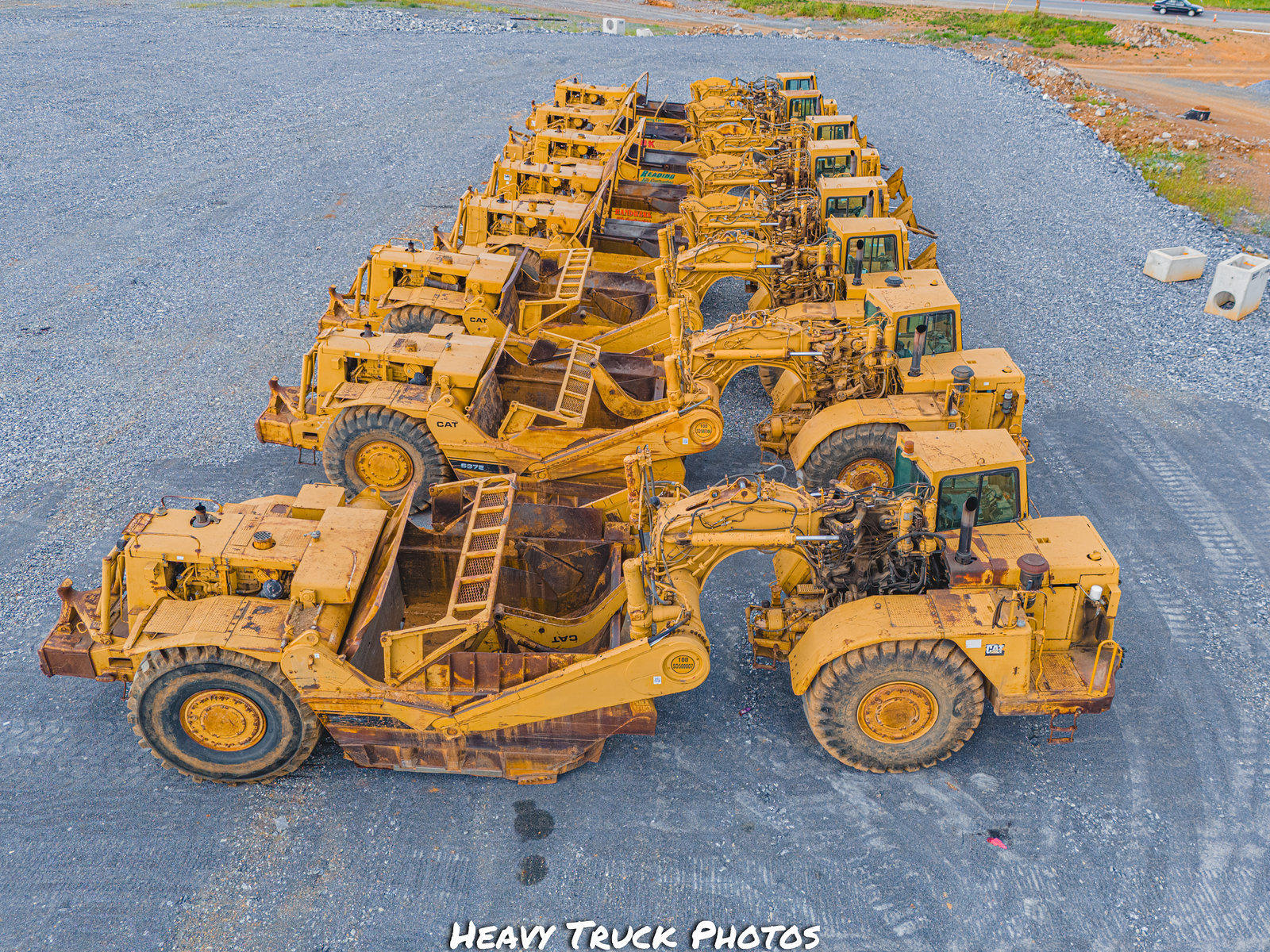The image captures a wide, leveled gravel lot on a sunny day, seemingly part of a construction site undergoing active development. Within this lot, a single row of eight yellow tractor-trailers, each towing sizable equipment, stretches across the frame, meticulously spaced about 50 feet apart. Dominating the scene, these machinery pieces are marked with the brand name "CAT" and equipped with large, thick tires featuring yellow rims. Each tractor-trailer is approximately 15 feet long, highlighting their considerable size compared to the smaller, less discernible car positioned in the background to the upper right. The lot itself is bordered with sporadic patches of dirt, grass, scattered sticks, and some cinder blocks, reinforcing the sense of an ongoing construction project. At the bottom center of the photo, the text "heavy truck photos" is prominently displayed in white.